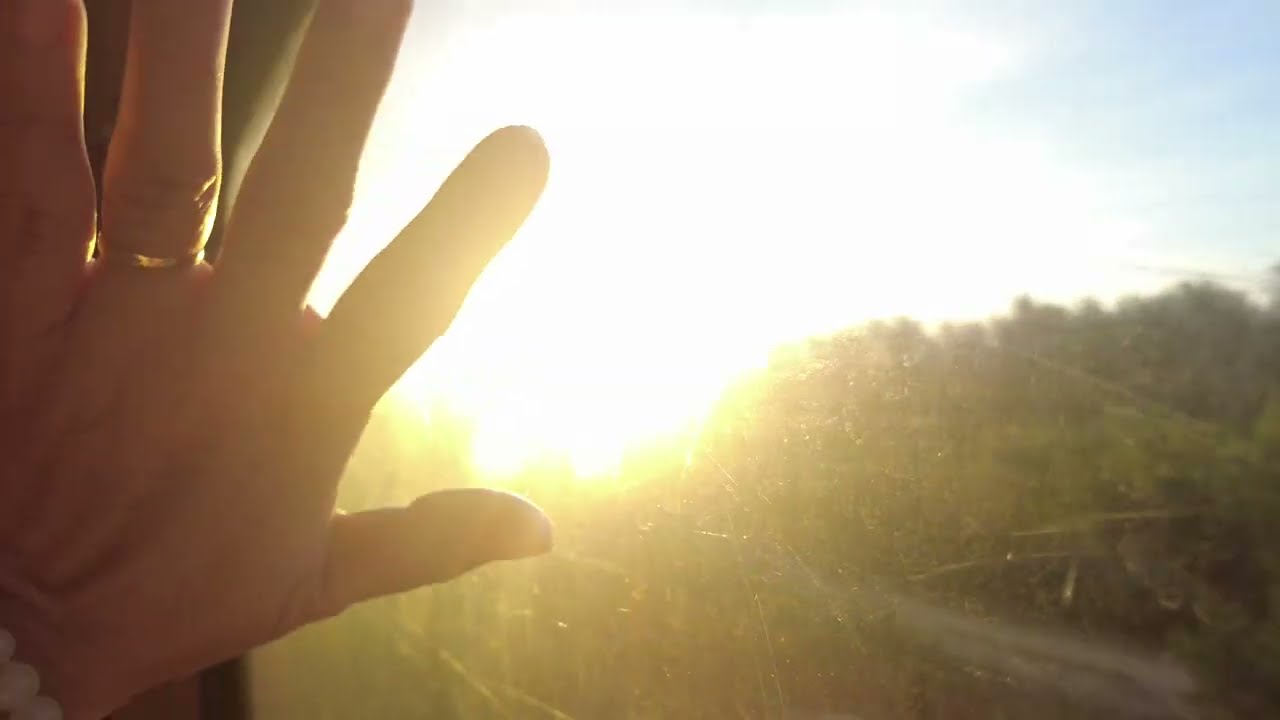The photograph features a prominently displayed hand on the left side, with fair skin and a golden wedding ring on one finger. All five fingers, as well as the palm, are clearly visible, and the hand appears to be spread as if signaling "stop" or "go back." The image is overexposed, contributing to the bright, glaring sunlight occupying the center, which floods the scene with white light. Behind the hand, the rest of the person's body is obscured by the brightness. To the right, the view is partially blurred but shows green trees and a blue sky transitioning to white in the middle, indicating the sun's intense presence. The overall composition suggests the photo was taken facing the sun, possibly through a window, perhaps during travel on a train or an airplane.